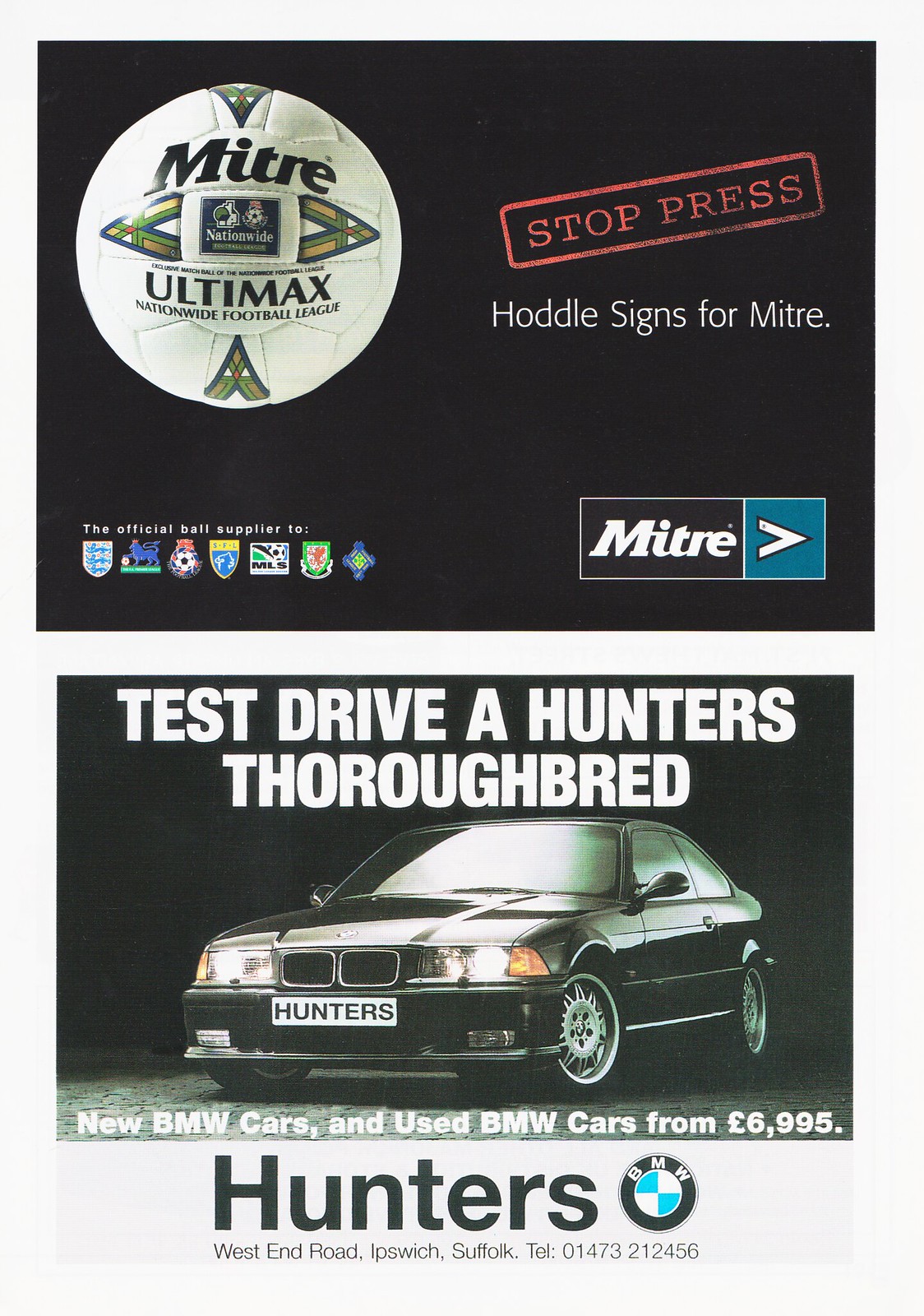The image showcases a digital screenshot of two distinct half-page magazine advertisements on a white background. The upper half of the page features an advertisement for the Mitre Ultimax soccer ball. Positioned within a black square, the upper left-hand corner prominently displays a white soccer ball labeled "Mitre Ultimax," accompanied by the text "the official ball supplier to" followed by several company logos. In the upper right-hand corner of the black square, the phrase "Stop Press" appears in bold red letters, with "Hoddle signs for Mitre" noted beneath it. 

The lower half of the page is dedicated to a car advertisement for BMW. Another black square contains the white text "Test Drive a Hunter's Thoroughbred." Directly below is an image of a sleek black BMW, featuring a license plate that reads "Hunters." The subsequent text promotes both new and used BMW cars starting from £6,995. The ad concludes with the dealership's name "Hunters" in red letters, alongside the BMW logo, and provides further contact details including the address "West End Road, Ipswich, Suffolk" and a telephone number.